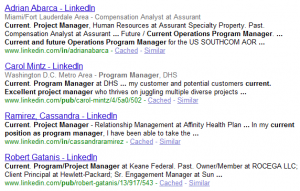Sure, here is a cleaned-up and highly detailed caption:

---

A screenshot of a Google search displaying various LinkedIn profiles in the search results page. The following details are included in the image:

1. **Adrienne Arbica**: Based in the Miami-Fort Lauderdale area, currently a Compensation Analyst at Ashrant with additional roles including a Project Manager in Human Resources for Assurance Specialty Property. Her past experience includes a role as a Compensation Analyst at Assurance, and she is slated to become an Operations Program Manager for the US Southern Command. Her LinkedIn URL is `www.linkedin.com/in/adriana-abacara`.

2. **Carol Mints**: Located in the Washington D.C. metro area, presently working as a Program Manager at the Department of Homeland Security (DHS). Her profile highlights her skills in managing diverse projects. Her LinkedIn URL is `www.linkedin.com/pub/carol-mints/4/5`.

3. **Cassandra Ramirez**: Currently a Project Manager specializing in Relationship Management at Affinity Health Plan. Her profile mentions that she has significantly contributed to her current role as a Program Manager. Unfortunately, the text cuts off after mentioning her current contributions. Her LinkedIn URL is `www.linkedin.com/in/cassandra-ramirez`.

4. **Cassandra Roberts**: Now a Project Manager at Keene Federal with a history as an Owner and Member at Rock Gaga LLC. She has held senior management roles including Client Principal at Hewlett-Packard and an executive position at Sun Microsystems, though the full details are truncated. Her LinkedIn URL is `www.linkedin.com/pub/roberts-cassandra/a string of numbers`.

Each entry also includes the words "cashed" and "similar" at the end, indicating that Google provides cached versions of these pages as well as links to similar profiles.

---

This detailed caption gives a comprehensive overview of the information visible in the Google search snapshot.